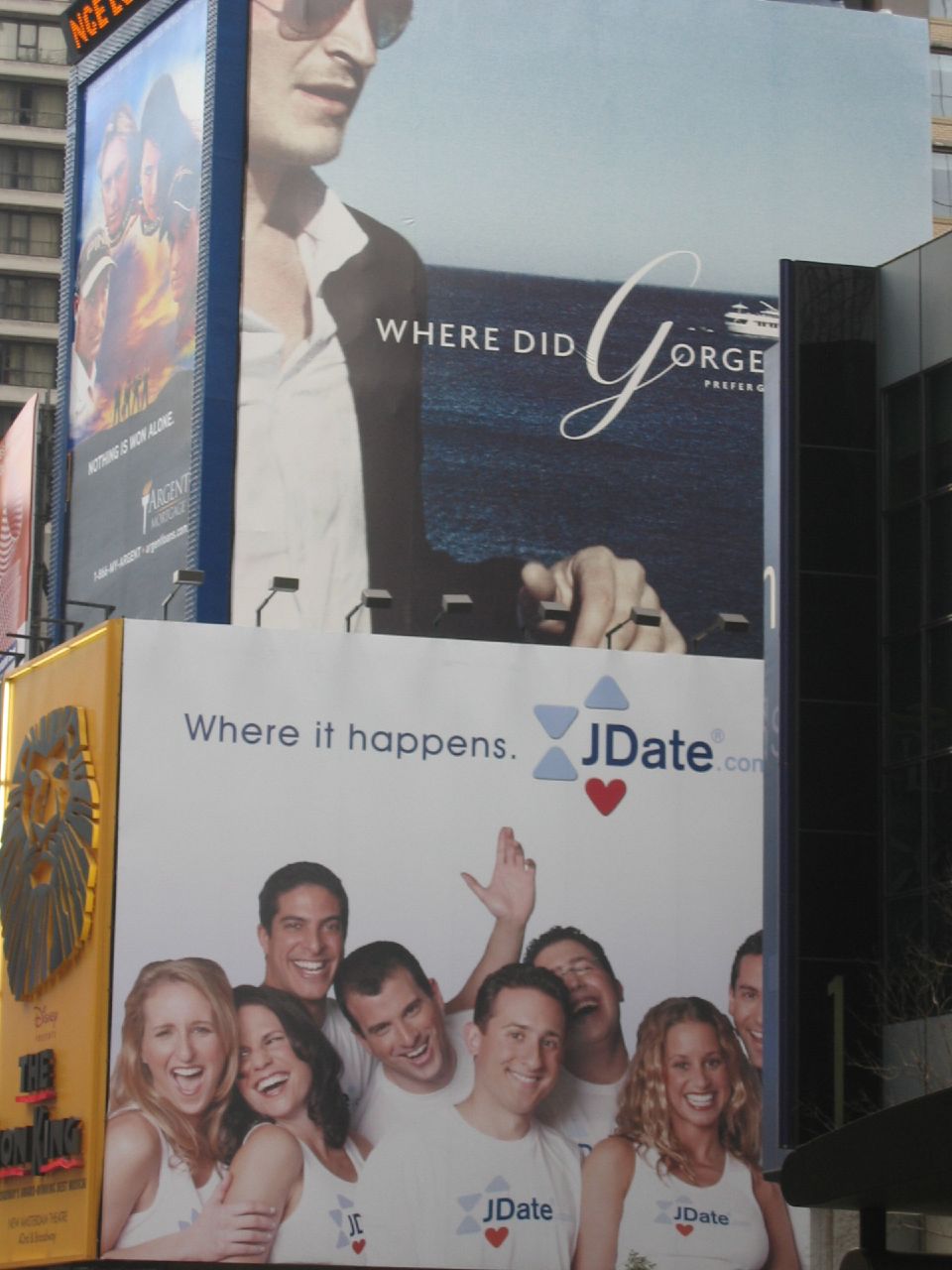This image showcases a vibrant building covered in numerous advertisements, reminiscent of the iconic Times Square in New York City, suggesting its possible location there. Dominating the lower center of the photograph is an advertisement for jdate.com, featuring several smiling individuals, both male and female, clad in t-shirts and tank tops emblazoned with the "jdate" logo. The text on this ad reads "Where It Happens," enhancing the community spirit depicted. Directly above this, another advertisement features a man donning sunglasses, set against a serene backdrop of the ocean with a boat visible in the distance. The intriguing text associated with this image reads "Where Did George?". Situated to the left of the jdate.com advert is a promotional display for the renowned musical "The Lion King."